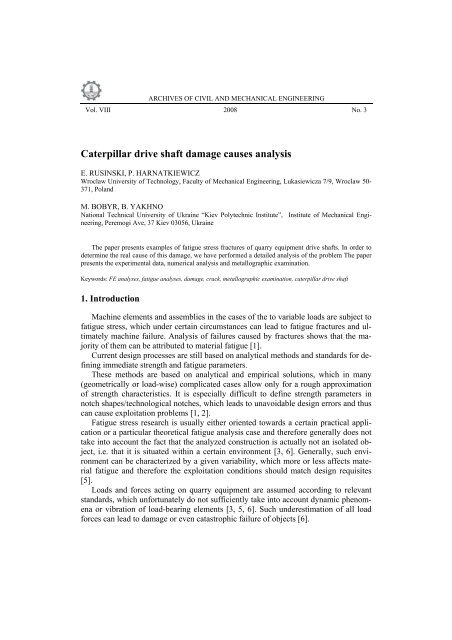This image depicts the first page of a scientific article titled "Caterpillar Driveshaft Damage Causes Analysis" from the *Archives of Civil and Mechanical Engineering*. The article is from Volume VIII, Number 3, published in 2008. The authors are E. Racinski and P. Harnackiewicz. The page, written in a standard typeface akin to Times New Roman, includes the title in bold at the top and is followed by an abstract and the beginning of the introduction section. The initial lines discuss fatigue stress in machine elements and assemblies, emphasizing that the majority of fractures result from material fatigue. The analysis covers the challenges in defining strength parameters, especially in geometrically complex or notched shapes, and underscores the inadequacy of current design standards in accounting for dynamic phenomena and vibration in load-bearing elements, which can lead to serious damage or failure. The resolution of the image is somewhat blurry, making the text difficult to read clearly.